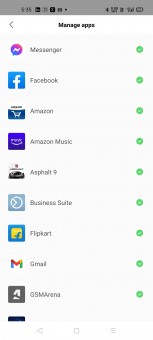Caption: 
A blurred screenshot displays a mobile app manager interface with the title "Manage Apps" clearly visible at the top in black font. Each app in the list has its respective icon positioned to its left, and a small neon green circle with a white checkmark situated to its right, likely indicating a selection or enabled status. The apps listed, presented in grey text, include Messenger at the top, followed by Facebook, Amazon, Amazon Music, Asphalt 9, Business Suite, Flipkart, Gmail, and GSM Arena.